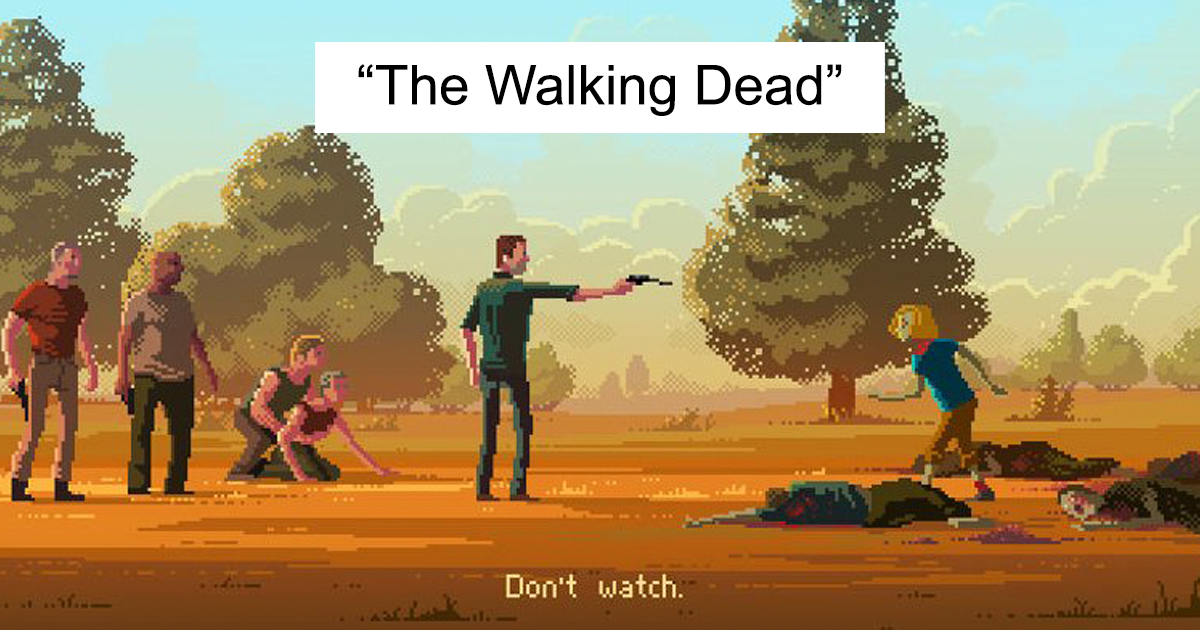The image is a pixel art illustration reminiscent of a video game, featuring a scene from "The Walking Dead." At the top of the image, a white rectangle with black text displays the title "The Walking Dead," while the bottom contains the phrase "don't watch" in white text. The setting includes a brown, soil-like ground with a backdrop of green trees, mountains, a blue sky, and white clouds.

In the center, a man in a green shirt and jeans points a pistol at a figure with shoulder-length blonde hair, wearing a blue shirt and brown pants. This figure appears to be a child or possibly a smaller person. Surrounding them, three bodies lie on the ground, bleeding, suggesting they could be zombies or deceased people.

To the left, a man in a red shirt and khakis stands apart from a heavier man with brown skin, donning a brown shirt and green pants. Behind the central figure with the pistol, a woman with short hair in a red shirt is kneeling, with a man in a green shirt and khakis, who has yellow hair, holding her around the waist. The entire group stands on an orange-brown ground, and the serene background contrasts with the intense foreground action.